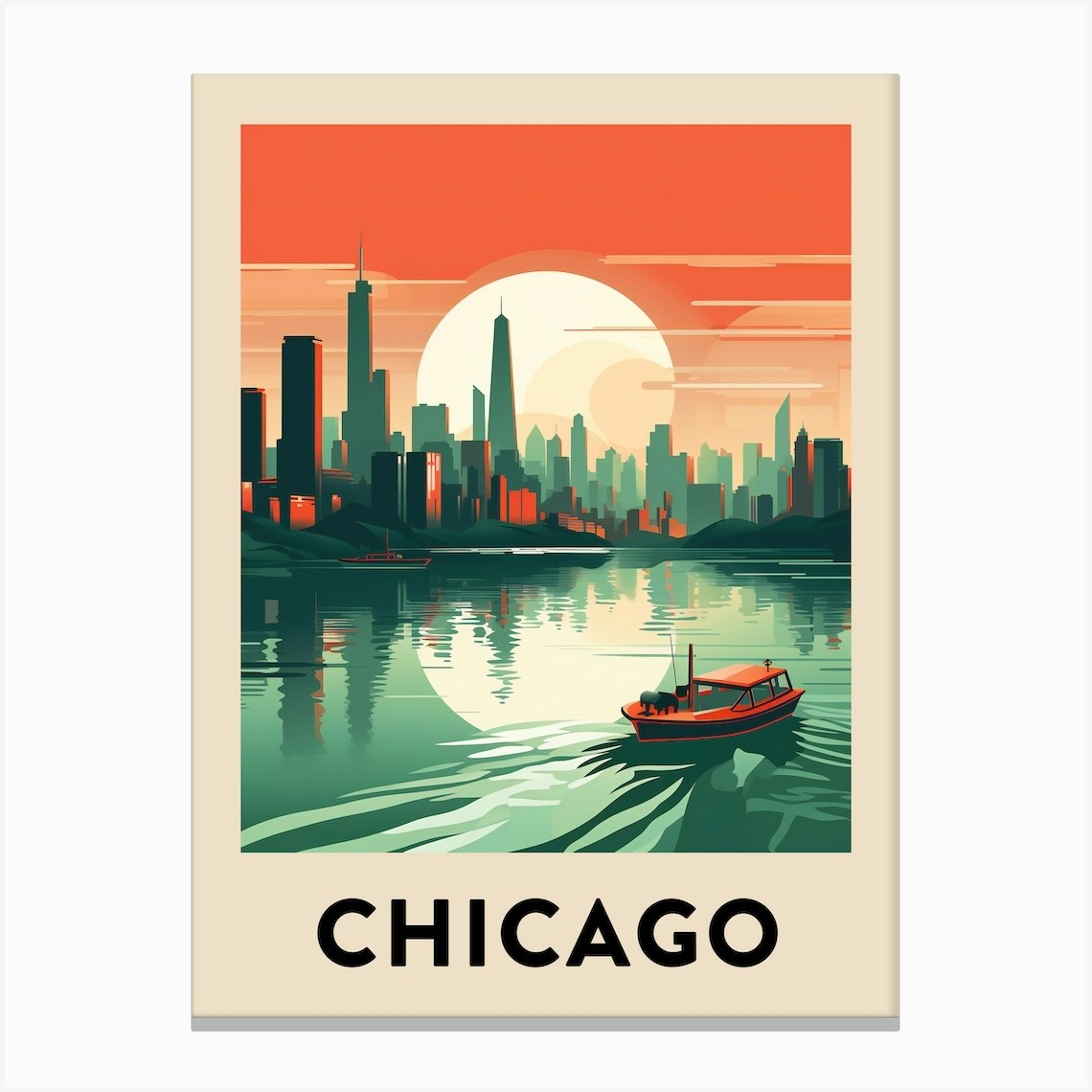The image is a detailed poster of the Chicago skyline, mounted on a white wall with a beige-colored border that is thicker at the bottom than on the other sides. At the bottom of the poster, in large black capital letters, it prominently says "CHICAGO." Above the text, there's a well-executed vector art illustration showcasing the city's skyline. Tall, needle-like buildings are situated on the left side, with the foreground structures in darker green and those farther away in pale green hues. A large white sun dominates the background, supported by stylized, light orange clouds with brighter orange tops. The upper half of the poster features an orange-red sky, indicating either a sunrise or sunset. In the lower half, green water reflects the white sun and cityscape. A red boat, likely a tugboat, steams towards the right, leaving a wake behind it. Along the shoreline, small houseboats are visible. Recognizable buildings such as one with a slanted roofline, possibly the Prudential Building, and a pyramid-shaped structure with a spire can also be seen against the vibrant sunset sky.